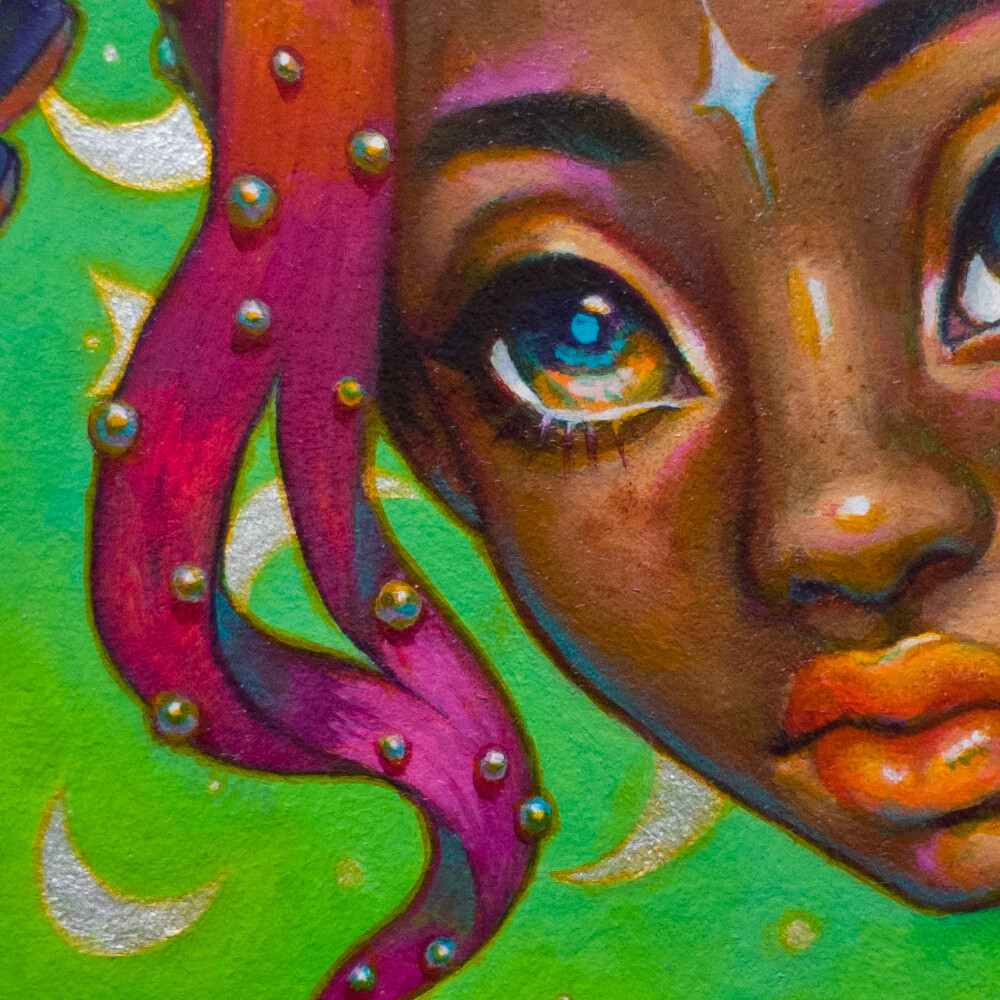The image is a close-up shot of a colorful painting, likely made with chalk or paint, featuring a dark-skinned female, possibly Black or Latina. Her striking red hair, which transitions into neon pink and orange shades, is adorned with small decorative glitter balls and white shiny pearls. The background is split diagonally with vibrant green hues and is embellished with silver moons outlined in gold and scattered gold dots, resembling stars. The woman has large, expressive eyes that transition from yellow at the bottom to blue at the top. A distinctive blue star is positioned between her eyebrows, and she has orange-reddish lips. Pink shading accentuates the areas above and below her brow line. The composition captures the left side of her face in detail, partially cutting off the right side, giving an intimate and focused view of her vivid features and intricate details.